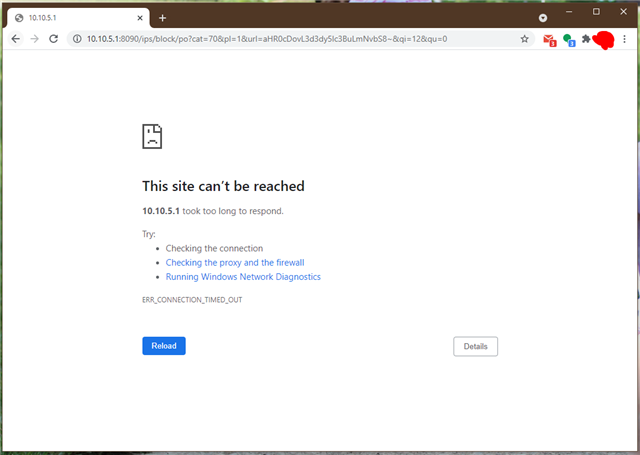This screenshot captures a Chrome browser with a single tab open, bearing the URL "10.10.5.1" and a globe icon, indicating a public site. The address bar at the top also displays "10.10.5.1". To the left of the address bar are navigation buttons, and to the right, there is a red bell icon with a "1" notification badge. Adjacent to this is a green icon with a blue number "3". Part of the user interface, likely the user profile avatar, has been obscured with red marker. The main browser window is stark white with a prominent message reading, "This site can't be reached. 10.10.5.1 took too long to respond." Below this message, three troubleshooting suggestions are listed in blue text:  "Checking the connection," "Checking the proxy and the firewall," and "Running Windows Network Diagnostics." At the bottom of the page, there are two buttons; a blue "Reload" button on the left and a "Details" button on the right.